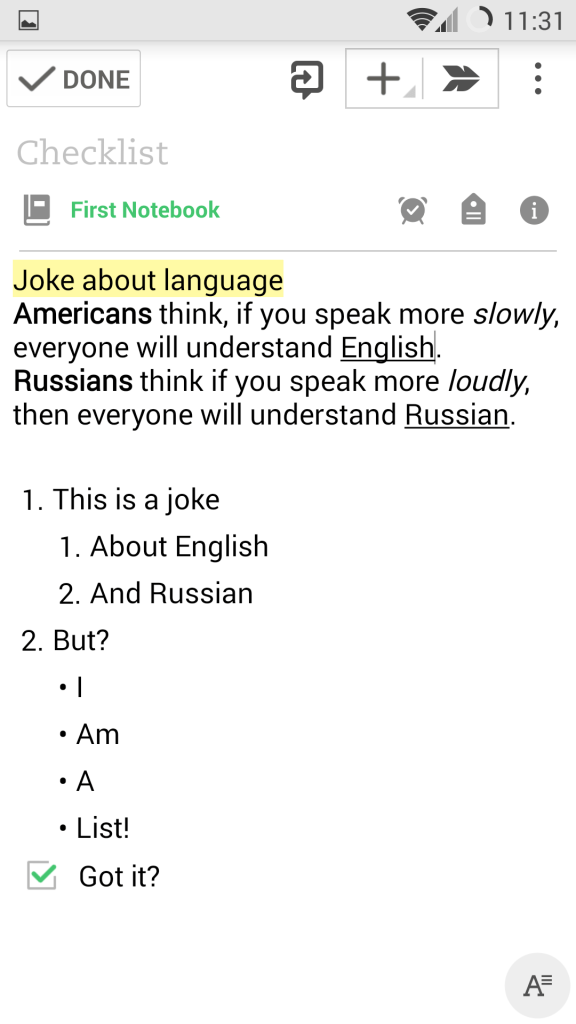A screenshot of a mobile device screen showcasing various interface elements against a white background. At the top-left corner, the screen displays a gallery icon, while the top-right corner shows a Wi-Fi icon and a connection icon, followed by the time "11:31." 

Directly below, on the bottom-left, there's a "Done" button accompanied by a checkmark. To the right of this, there are three icons: a plus (+) symbol, and three vertical dots. Beneath these, in a gray font, is the word "Checklist." Underneath this is the label "First Notebook" in green.

On the right side of the screen, there are icons for a clock, a house, and an eye. Centered on the screen, highlighted in yellow, is the text "Joke about language" in black. Below this, more black text reveals a humorous observation: "Americans think if you speak more slowly everyone will understand English. Russians think if you speak more loudly everyone will understand Russian." 

The content includes numbered jokes: "Number one, this is a joke," followed by "Number one about English," and "Number two in Russian" with a question mark. There are five notes listed vertically, with the bottom one stating "Got it?" Next to it is a square with a green checkmark. At the very bottom of the screen, there's a light gray circle containing the letter "A" next to an equal sign. The entire interface is set against a clean, white background.